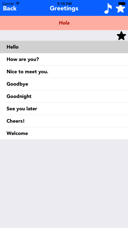The image appears to be a screenshot from a mobile device, characterized by a royal blue border at the very top. On the left side of this border is a back button, while the middle portion prominently displays the text "Greetings." To the right, there are two icons: a music note and a white star. Above the "Greetings" text, though somewhat blurry, the time can be partially discerned, showing the letters "PM." Below this section, a reddish background briefly appears, with the word "hola" in white text on it. 

This reddish section is bordered at the bottom by a gray strip that features a black star on the right side. Below it, there is a gray bar displaying the heading "Hello." Underneath this heading, a list of greeting options extends downward in a column. The options include "How are you," "Nice to meet you," "Goodbye," "Good night," "See you later," "Cheers," and "Welcome." It's evident that the option "Hello" has been selected by the user. At the very bottom of the screen, a large gray rectangle occupies the remaining space, indicating that this section is empty or not relevant to the greeting options displayed above.